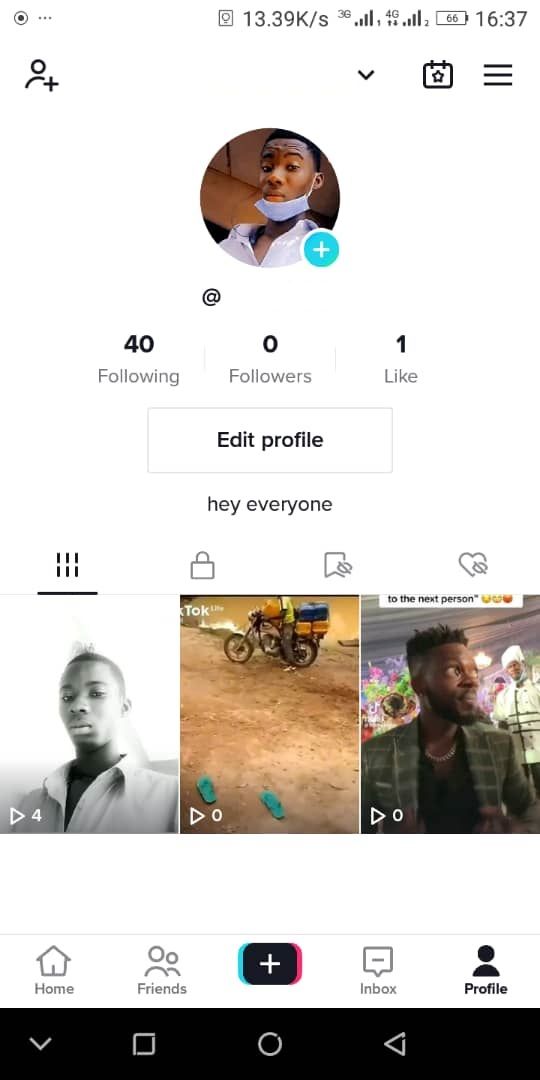This screenshot captures an intricately detailed view of a TikTok user’s profile page, taken from a smartphone. Starting from the top-left and moving across, there is a small circle icon accompanied by a dark-filled circle, possibly indicating a screen recording app. Adjacent to it, there is an ellipses icon of unknown functionality, followed by an indeterminate square icon with a circle in its center. Next, there is text displaying “13.39K/s,” likely denoting some network speed metric. Further right, indicators show both 3G and 4G connections at full bars, a battery level, and finally, the current time, enriching the top status bar with comprehensive details.

Below this, the TikTok profile page becomes the focus. On the top-left, a small person icon with a plus sign signals an option to add friends. Moving right, a dropdown arrow likely provides friend suggestions, followed by a calendar icon with a star, perhaps for checking dates like birthdays. Further to the right, a hamburger menu provides more options.

Centralizing onto the true content, the profile picture shows an African-American man wearing a blue shirt with a mask pulled down to his chin. An overlay icon with a plus sign suggests an option to change this profile picture. Below, his username is obscured by whiteout, yet visible metrics for “Following,” “Followers,” and “Likes” are displayed. An “Edit Profile” button is positioned beneath these stats. Below this, his bio reads, “Hey, everyone.”

The lower section features four distinct tabs for organizing content: Posts (represented by a grid icon), Locked Posts (with a lock icon), Hidden Bookmarks (ribbon with an eye through it), and Hidden Hearts (heart with an eye). Beneath these tabs are three video thumbnails depicting his recent TikToks.

The navigation bar at the bottom includes icons for Home, Friends, a central Creation button for making TikToks (depicted as a rectangle with a plus), an Inbox for messages, and the User Profile. Further down, the smartphone's standard navigation bar includes a down arrow, a square to access other apps, a circle for the home screen, and a back triangle to navigate backwards. 

The composition of this screenshot not only provides a detailed overview of the TikTok profile but also captures the multifaceted interface of the smartphone in use.